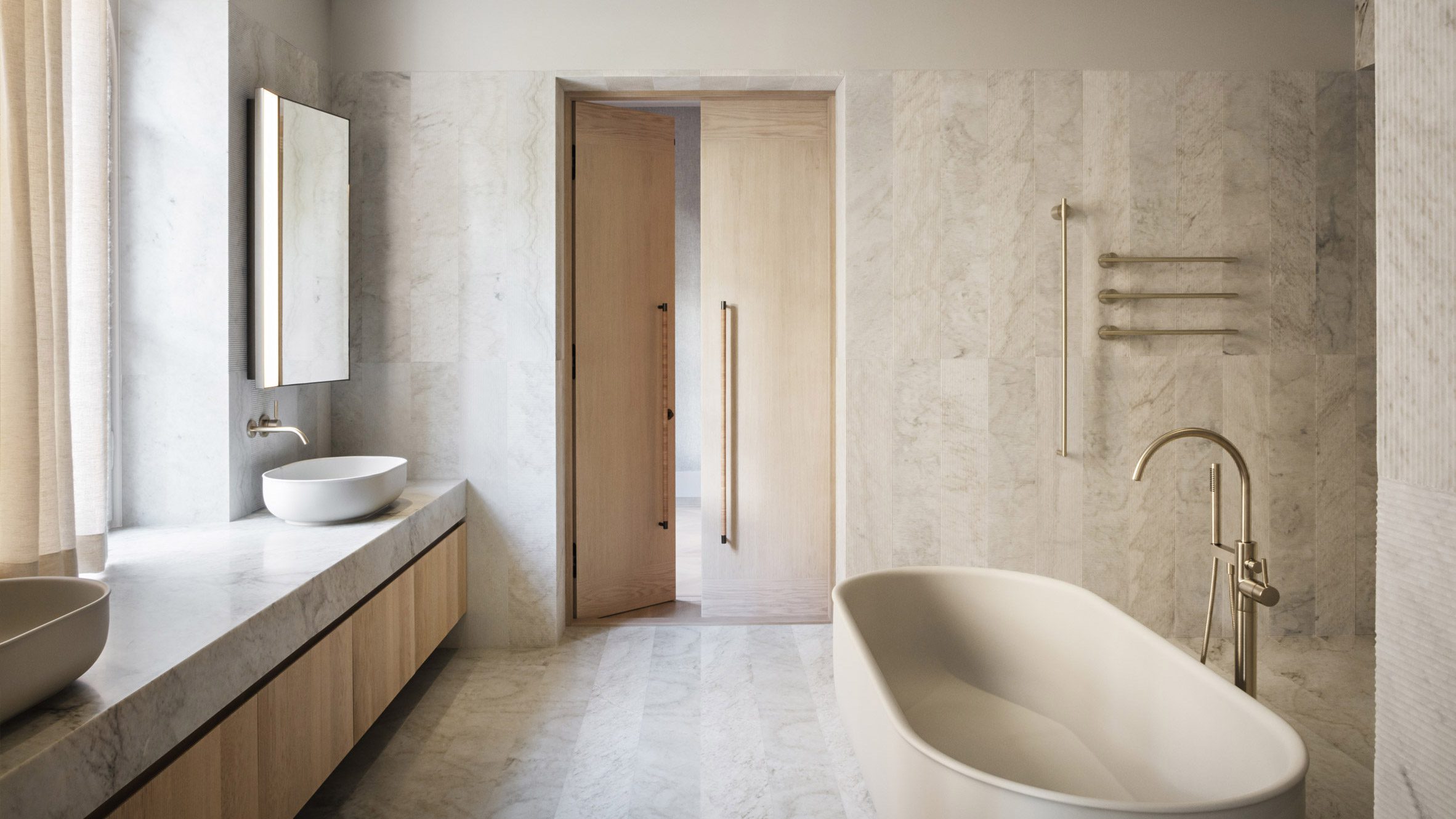The photograph captures the serene elegance of a modern, minimalist bathroom bathed in daylight. The room exudes a cohesive design with light gray stonework adorning the floor, walls, and the expansive countertop on the left. The countertop houses two oblong, round, raised white basins, with a sleek wall-mounted faucet in between. Beneath this counter lies a light brown wooden cabinetry providing ample storage.

On the left-hand side, there is a wide window framed by light brown curtains that allow soft white light to filter through, brightening the space. Above the faucet area, a medicine cabinet, possibly mirrored, adds a practical touch to the setting.

The back center of the image reveals double wooden doors, finished in a light brown hue. The door on the right remains closed while the one on the left stands ajar. To the right, the walk-in shower area appears open and accessible, seamlessly integrating into the overall design. In front of the shower, a sleek, elongated elliptical white bathtub features prominently. It is complemented by a stylish, raised silver faucet behind it, arcing gracefully from the floor.

Steel hangings on the wall serve as multifunctional towel racks, some perhaps incorporating lighting elements for added functionality. The meticulous blend of materials—marble-like countertops, granite floors, light wood furnishings, and steel fixtures—creates a harmonious and ultra-modern aesthetic.